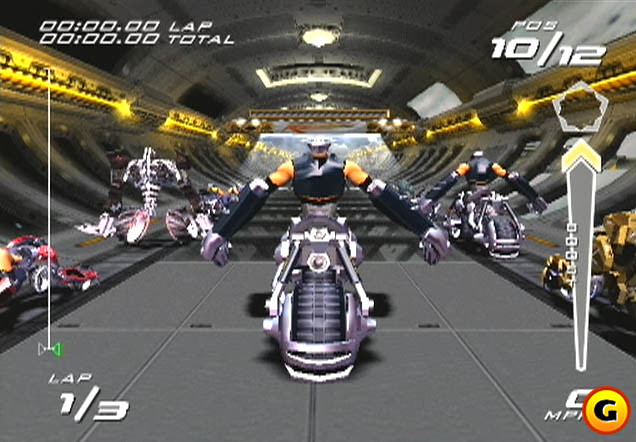The image is a detailed screenshot from a racing video game set in a steel tunnel that extends into the distance. The scene is predominantly gray, broken up by yellow laser-like lights along the sides of the tunnel and glass tubes containing a central yellow laser. In the foreground, a large, imposing robotic figure with an intricately detailed metal head and enormous arms sits atop a futuristic motorcycle with a robust steel frame and a prominent fat front tire. This figure, facing towards the viewer, is adorned in black arm sleeves and purple-silver gloves. Surrounding this central character are numerous similar robotic vehicles, all lined up and prepared for the race.

The interface displays typical racing game metrics: on the bottom left, it indicates "Lap 1 of 3," while the bottom right corner shows a yellow circle with a red border and a black capital 'G,' partially obscuring the speedometer that reads "0 MPH." The top right corner shows the current position as "POS 10/12," and the top left lists the lap time and total time as "00:00.00 lap" and "00:00.00 total" respectively. The overall ambiance suggests a high-stakes racing scenario, with the possibility of encountering other competitors or obstacles within the tunnel's depths.